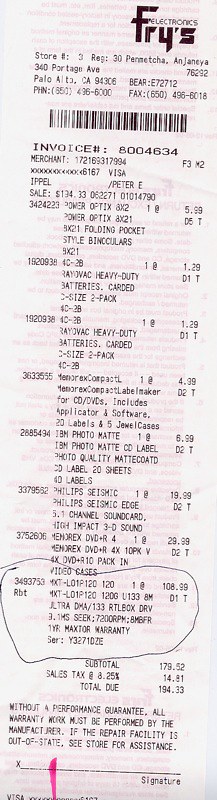This is a photograph of a receipt from Fry's Electronics, located at 340 Port Aguayo, Palo Alto, California. At the top of the receipt, the store name and address are prominently displayed, followed by the store's phone number and fax number. A section labeled "BEAR" (possibly an internal code) is accompanied by a number beginning with the letter "E." Below this, a barcode is visible, and the invoice details including the invoice number are listed. The receipt then itemizes the purchases, with one particular section near the bottom noticeably circled, drawing immediate attention. This circled section includes an item marked with "R-B-T" and a corresponding price of $108.99 on the right side. The receipt is densely packed with various numbers, abbreviations, and letters, making it somewhat difficult to discern the exact details of the purchases, though it may potentially involve video cases. Despite being in English, the technical nature of the receipt poses challenges for those unfamiliar with electronics and related terminology.